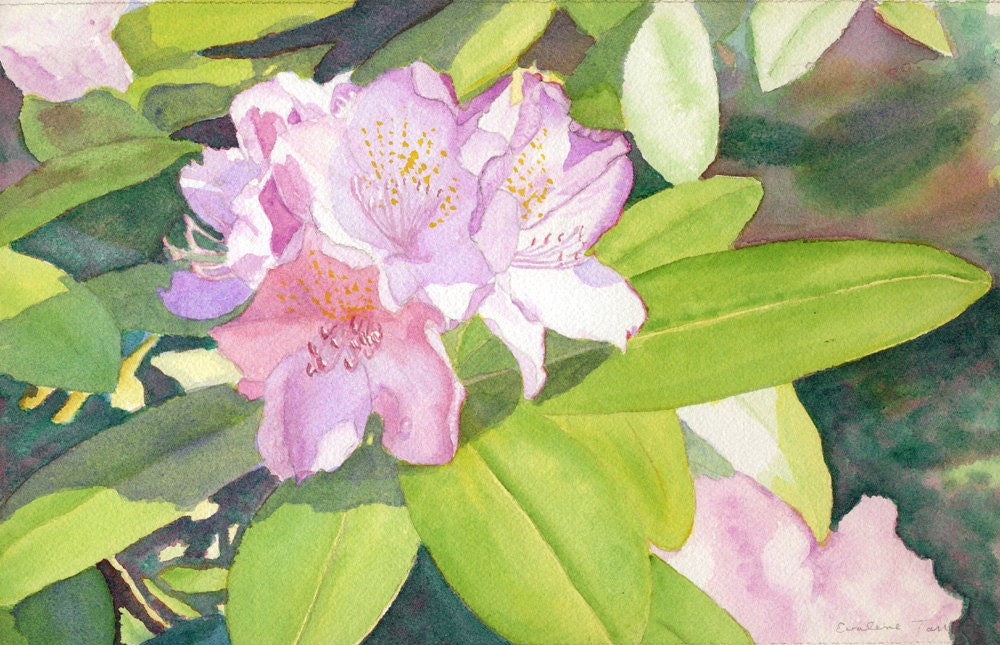This is a detailed watercolor painting depicting clusters of flowers and elongated, oval-shaped leaves. The green leaves prominently feature yellow centers, veins, and subtle threading. The flowers themselves have webbed, star-shaped petals, rendered in light pink with hints of white and purple. Each flower's center boasts rich golden-orange pollen, with some displaying yellow and red dotted structures. Variations in blue, brown, pink, and purple hues fill the background, alongside notable dark brown shades, adding depth to the composition. Notably, there is no presence of animals, insects, or any text. However, a small, barely legible black initial appears in the bottom right corner. The overall artwork is a vivid display of botanical beauty, focusing fully on the interaction between the flowers and leaves.